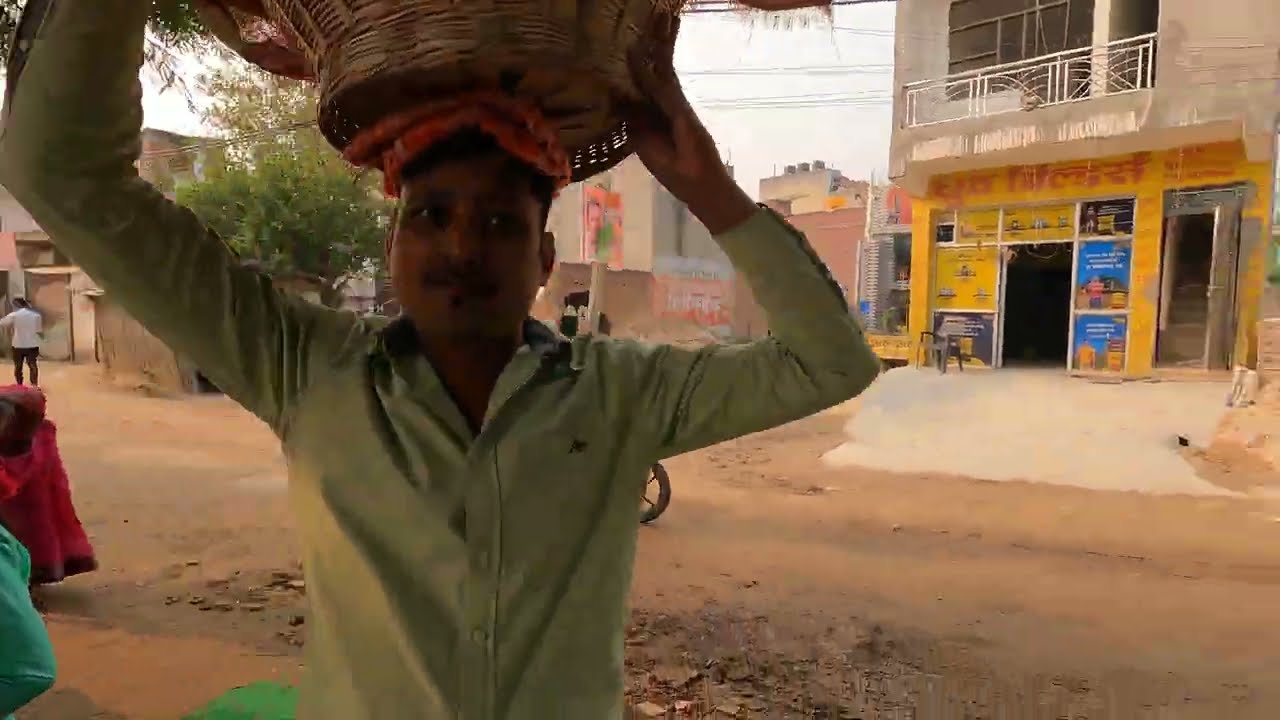In the landscape photo, a dark-skinned Indian man, dressed in a mint green long-sleeved button-up shirt, is positioned centrally and captured from the waist up. He carries a large, circular, cream-colored woven basket on his head, securing it with both arms while looking straight into the camera with a neutral expression. The dirt road he stands on is framed by a series of colorful, old buildings, suggesting a remote but potentially busy city area. To the right, a yellow building with an open door and signage in yellow, blue, and black adds a splash of color. A chair is visible just outside this building. Behind him, to the left, a tree stands tall, with a person partially visible in black pants and a white shirt. Overcast skies and electric wires loom above, contributing to the rustic ambiance of the scene. A bicycle and a couple of people are also faintly visible in the background, further hinting at the local activity.